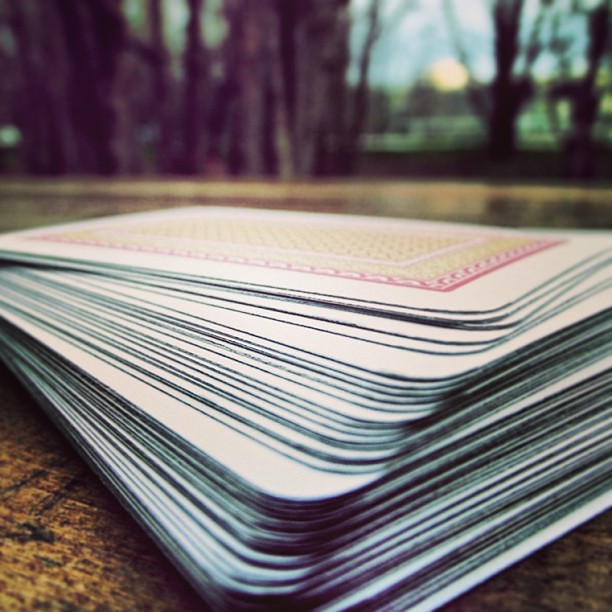This photograph captures a close-up view of a stack of playing cards precariously leaning as if they're about to topple over. The cards rest on what appears to be either a wooden floor or a brown carpet, though it could also be a table. The background is heavily blurred, showcasing indistinct but recognizable elements like trees, grass, sky, and sunlight, suggestive of a woodland scene. The image exudes a nostalgic, 1970s vibe, emphasized by its limited and muted color palette. A bluish-purplish tint enhances the vintage aesthetic, reminiscent of old-fashioned photography. Notably, the photograph is a perfect square, a rare format in contemporary photography, further amplifying its retro appeal. The playing cards themselves have yellow backs with a red border, appearing to form a complete set, though their exact number is indeterminate. Their arrangement suggests a casual toss onto the surface.